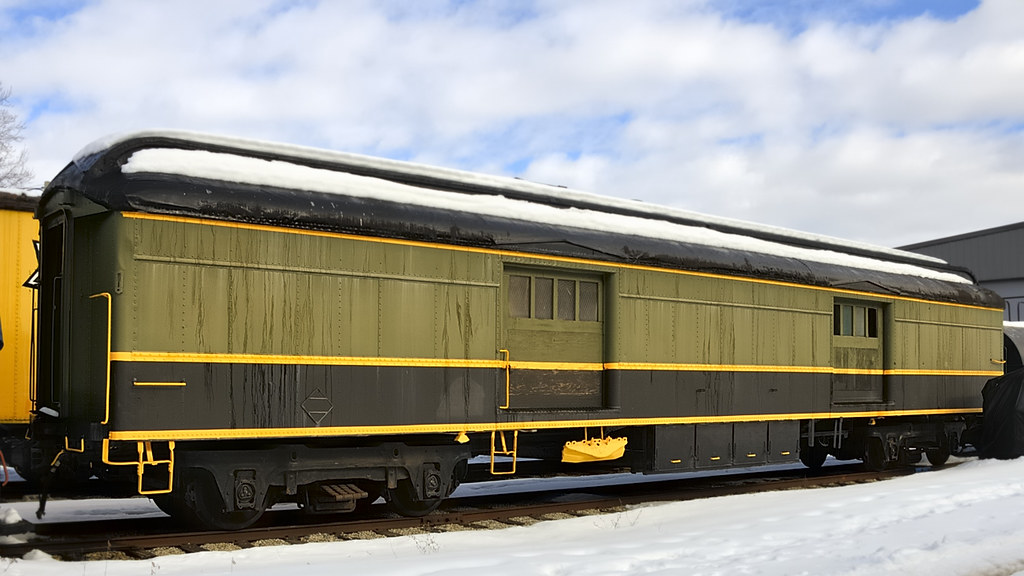This photograph captures a detailed and well-maintained freight train car, bathed in a serene, snowy setting. The train car, dominating most of the image, is primarily a dark, army green color accented by bold yellow trim and steps, as well as yellow handles and stripes that run along its length. The car's design features prominent sliding doors reminiscent of barn doors or industrial factory doors. The lower section of the train car is black, accented with bright yellow highlights. Snow blankets the ground beside the tracks and delicately dusts the top of the train, suggesting a recent snowfall. In the background, partially visible is a second train car painted in a bright yellow hue. The scene unfolds under a partly cloudy sky with patches of blue peeking through, adding to the overall calm and picturesque atmosphere, indicative of a possibly preserved location such as a museum. The entire setting hints at a beautiful, tranquil day, with a vintage, yet well-kept railcar at its heart.